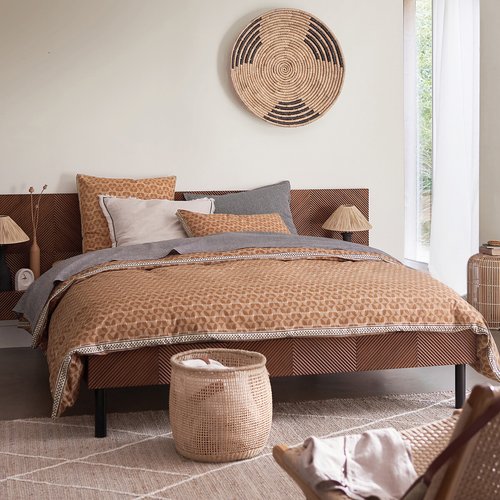The photograph depicts a well-appointed bedroom with a central theme of beige, brown, and gray tones. The queen-size bed, positioned against a cream-colored wall, features a dark brown cushioned headboard. It is adorned with pillows in shades of gray and cream, along with a folded-back quilt showcasing a leopard print motif in brick red on a cream background. Below this comforter lies a gray sheet, adding another layer of texture and warmth.

On the wall above the bed, there is an artistic round wicker decoration in cream and black, contributing to the room's earthy aesthetic. Flanking the bed are two matching side tables, each with a small lamp providing balanced illumination.

At the foot of the bed sits a wicker clothes basket, adding both functionality and style. Supporting the bed are dark brown footstools. The floor features a tan rug with white stripes, enhancing the cozy atmosphere of the room.

In the bottom right corner of the image, a partially visible wicker chair with a wood frame and cream-colored woven pattern aligns with the room's overall design scheme. The vantage point of the photograph is from the front of the room, capturing the harmonious and inviting decor from this perspective. Additionally, there’s a large window to the right, partially covered by a white sheer curtain, allowing natural light to gently illuminate the space.